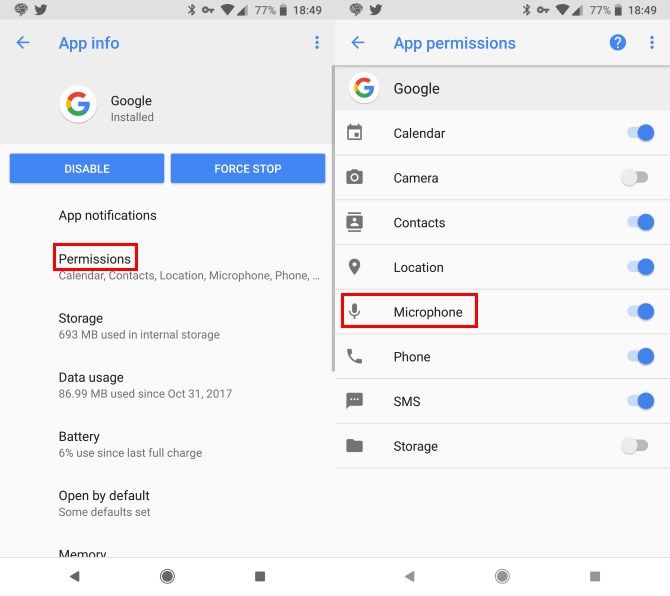The image captures a split-screen view of a smartphone interface displaying app information and permissions for the Google app. 

**Left Image:**
- A grey banner spans the top, showing system icons including a chat bubble, Twitter icon, and Bluetooth on the left, with Wi-Fi, network strength, battery level (77%), and time (18:49) on the right.
- Below the banner, the text "App Info" appears in blue font with a left-pointing blue arrow.
- Below, there's a white circle featuring a colorful 'G' for Google, labeled "Google installed."
- Two blue buttons underneath read "Disable" (left) and "Force Stop" (right).
- Further down, a list shows: "App notifications," "Permissions," "Storage," "Data usage," "Battery," "Open by default," and a partially visible "Memory."
- The word "Permissions" is highlighted with a red rectangular box.

**Right Image:**
- The top section echoes the left image, displaying "App permissions" in blue with a left-pointing arrow.
- Below, a blue banner showcases the Google logo and the word "Google."
- The app permissions are listed: Calendar, Camera, Contacts, Location, Microphone, Phone, SMS, and Storage.
- Blue or grey dots appear on the right side, indicating the status (on/off) of each permission.
- The word "Microphone" is highlighted with another red rectangular box.

This detailed composition showcases the user navigating app settings, emphasizing Permissions and the Google app's configurations.